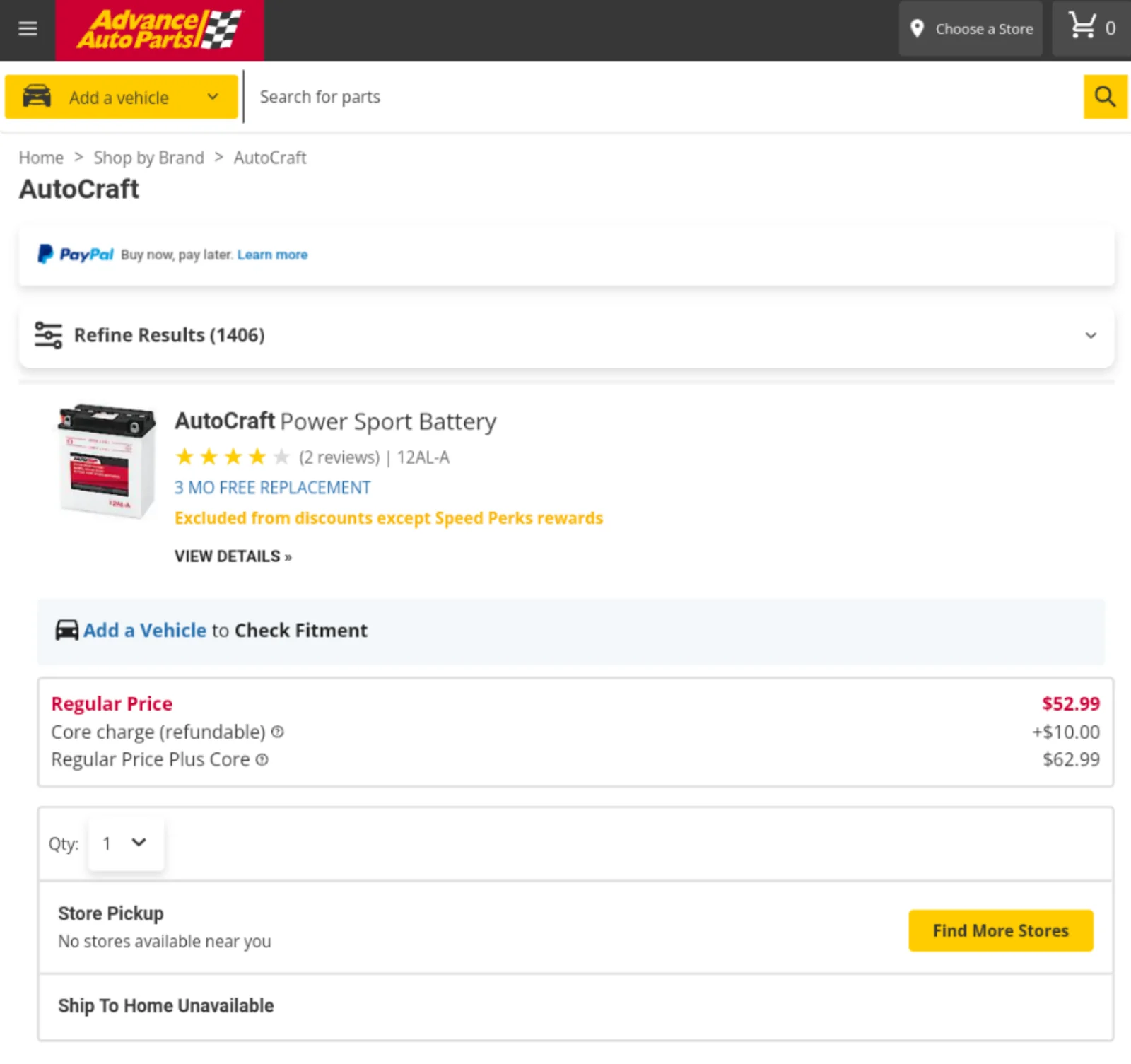This is a detailed and clean descriptive caption for the image:

---

The image depicts a webpage from the Advanced Auto Parts website. The website's branding is clearly visible in the top left corner, showcasing a red rectangular box with 'Advanced Auto Parts' written in yellow text. Adjacent to the text is a black and white checkered racing flag, all encased within a black rectangular box. The remaining background of the webpage is predominantly white.

Centrally located on the left side of the image is a picture of a battery. The battery has a white body with a black top and features a black and red label with information on the front. To the right of the battery image, the product is identified as the "Autocraft Power Sport Battery," which boasts a four-star rating out of five.

Beneath the battery image, towards the lower part of the webpage, the pricing details are presented. The regular price of the battery is listed as $52.99, with an additional refundable core charge of $10. This brings the total regular price plus the core charge to $62.99. The descriptions of the prices are conveniently placed to the bottom left, while the actual prices are positioned to the bottom right.